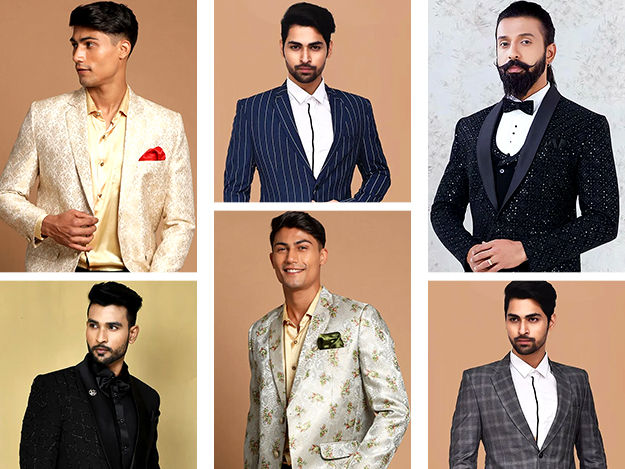The image displays a collection of six photographs of male models, each exuding elegance in their distinct suits, arranged in a horizontal rectangular layout. The top row comprises two rectangular photos and one square photo, while the bottom row includes one rectangle and two square photos. These sophisticated models, possibly Indian, vary in their facial hair: two have dark hair and mustaches, two are clean-shaven with dark hair, and two sport beards. The attire showcased ranges from a golden shiny coat with a diamond pattern and a red handkerchief in the top left to a black suit paired with a black shiny bow tie in the middle left. In the bottom middle, a model dons a silver shiny coat with green file patterns, accessorized with a green handkerchief, while the bottom right features a white and gray checkered pattern jacket over a white shirt with a central black line. The backgrounds feature soft colors like orange, peach, yellow, and white, enhancing the luxurious feel of the ensemble, making these men appear as if they could be movie stars or high-end models.